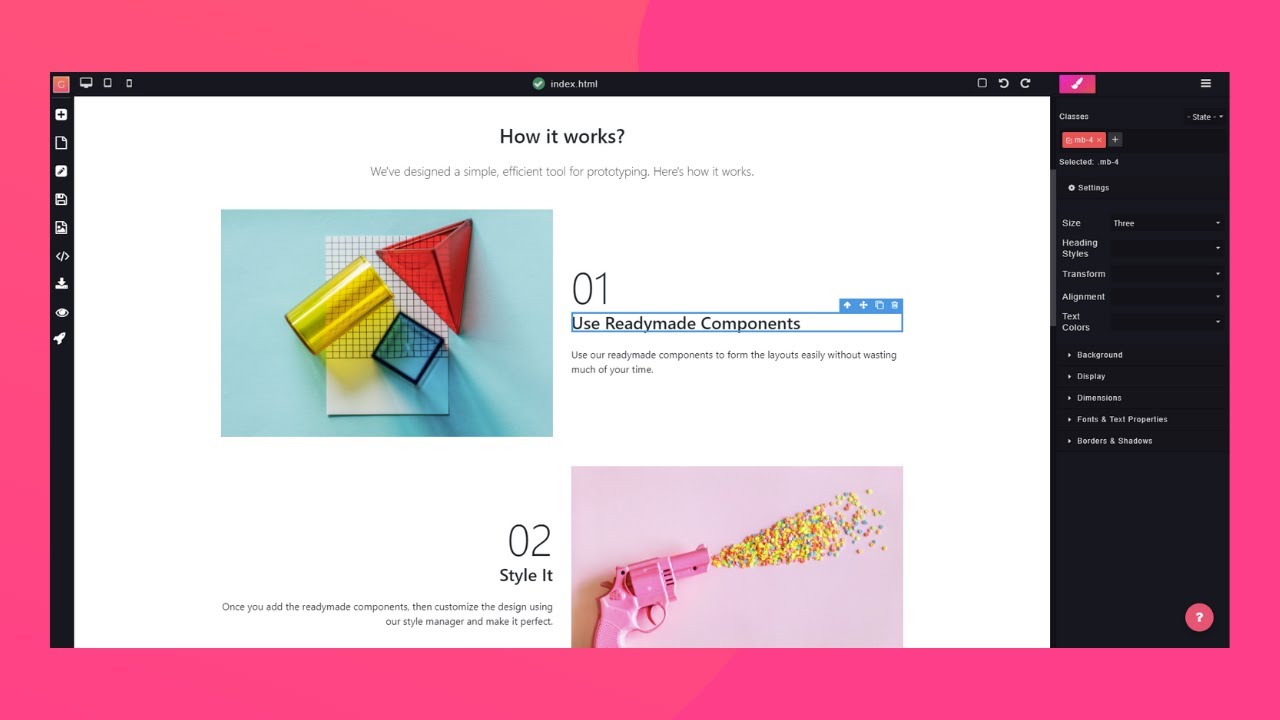This image is a detailed representation of an intuitive and efficient prototyping tool, emphasizing how simple and effective design creation can be.

At the top of the image, a header clearly displays a green circle with a white checkmark, labeled "index.html." The entire border of the section is red, drawing attention to its contents. Within this red-bordered section, there is a black frame enclosing a white background.

In the white section, the title "How it works?" is boldly written in black at the top. Below it, the text explains, "We’ve designed a simple, efficient tool for prototyping. Here’s how it works." The process is broken down into steps.

1. **Use Ready-Made Components**: This step encourages users to form layouts effortlessly using pre-made components, minimizing time spent on design. To illustrate, a picture on the left side shows a triangle, a cylinder, and a square object on a piece of paper against a blue background.

2. **Style It**: This step guides users to customize their designs with a style manager, perfecting the final look. The illustration for this step features a small pink gun shooting out colorful balls or candy-like pieces.

On the right side of the image, a vertical black rectangle houses various styling options:
- **Classes, State**: MB-4X is selectable with an add button.
- **Settings**: Features an icon for settings and options like Size 3 with a pull-down menu.
- Additional pull-down menus include Heading Style, Transform, Alignment, Text Colors, Background, Display, Dimensions, Fonts, Text Properties, and Borders and Shadows.

All these options are written in white, making them clear and easy to read against the black background.

To the left side of the image, additional icons are visible at the border, which features a thin black line. The top portion also contains various icons along with a paintbrush logo, indicating creative design tools.

This detailed and structured layout effectively demonstrates the ease and utility of the prototyping tool, guiding users through every step of the design process.